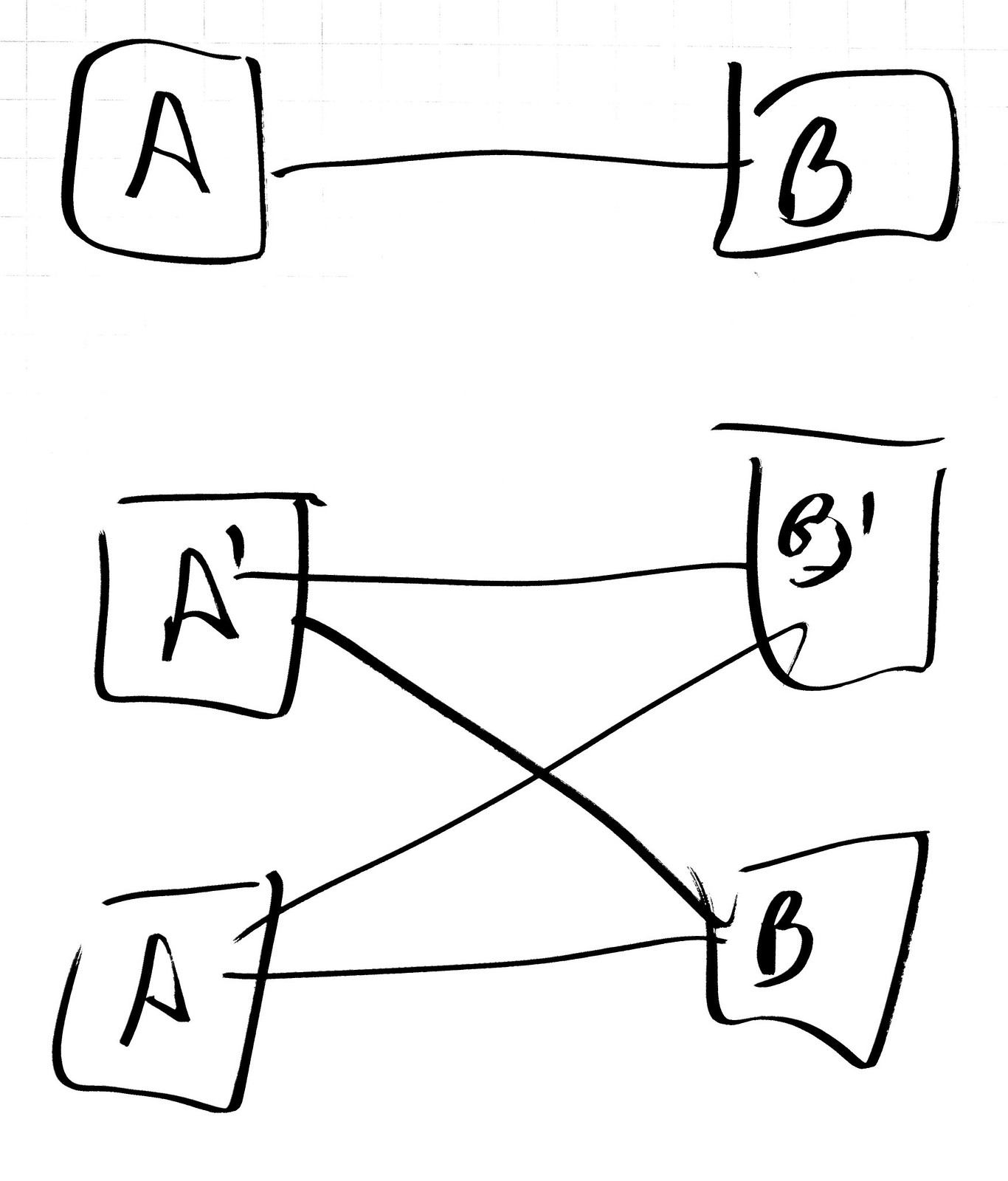The image features a meticulously hand-drawn diagram, likely created using a sharpie pen, set against a clean, white background. The diagram consists of six squares, strategically arranged and labeled. 

At the top, there are two squares labeled "A" and "B," each connected by a single horizontal line. Below these squares, there are four more squares arranged in a two-by-two grid. The squares in this grid are labeled "A'", "B'", "A", and "B" respectively. Specifically, the top-left square is labeled "A'", the top-right "B'", the bottom-left "A", and the bottom-right "B".

The diagram features several connecting lines: from "A" (top) to "A'" and "B'", from "B" (top) to "B'", and from "A'" to "B". The connections are drawn such that there are four interconnecting diagonal lines but no vertical lines connecting the "A" to "A'" or "B" to "B'".

Overall, the diagram appears to represent a structured, interrelated set of entities or concepts, meticulously connected to highlight relationships between them.